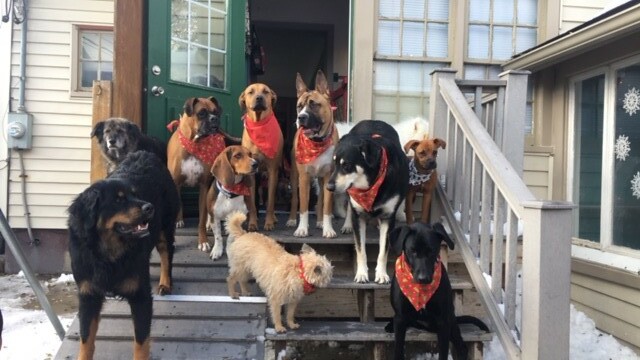This is a detailed colour photograph capturing a lively scene of numerous dogs gathered on a wooden staircase and ramp outside a house. The steps are grey and the accompanying ramp, which runs alongside, has black stripes and a silver spot. On the right of the steps is a grey handrail. The building behind the dogs is made of pale beige wooden planks, with a dark green door that is open, leading inside. The upper half of the door features a window pane, and there are more windows with white-painted frames on both the main building and a perpendicular section to the right. Notably, a large square window on the right has three white decorative snowflakes. Snow is visible on the ground around the steps and ramp.

The central focus of the photograph is the group of dogs. There are approximately 10 to 11 dogs present, ranging in size and breed, with a mixture of black, white, beige, brown, and tan coats. Each dog is adorned with a bandana, predominantly red, although there are exceptions with black and white bandanas. The dogs are various breeds, including larger ones like Labrador retrievers and smaller, fluffier breeds. They stand or sit on different levels of the steps and ramp, all facing different directions, capturing a moment of charming, organized chaos.